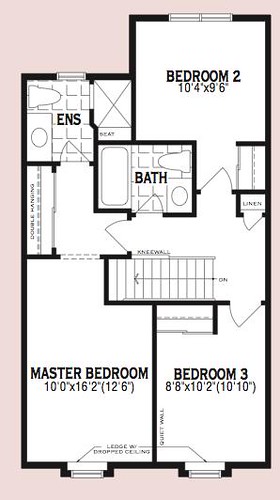This is a detailed house plan rendered using computer software with a pinkish background. The plan features black lines that delineate the structures and layout of the home. The primary structure is a large rectangle with a smaller rectangular extension. The interior includes a master bedroom and two additional bedrooms, each with its own window—two windows in one of the bedrooms and one in each of the others. 

There are two bathrooms, each equipped with a bathtub, toilet, and sink, all indicated by simple outlines. A centrally located staircase, depicted by a series of parallel black lines, descends to another level. The plan is represented in a black-and-white line drawing format, providing a clear and precise overview of the part of the home design.